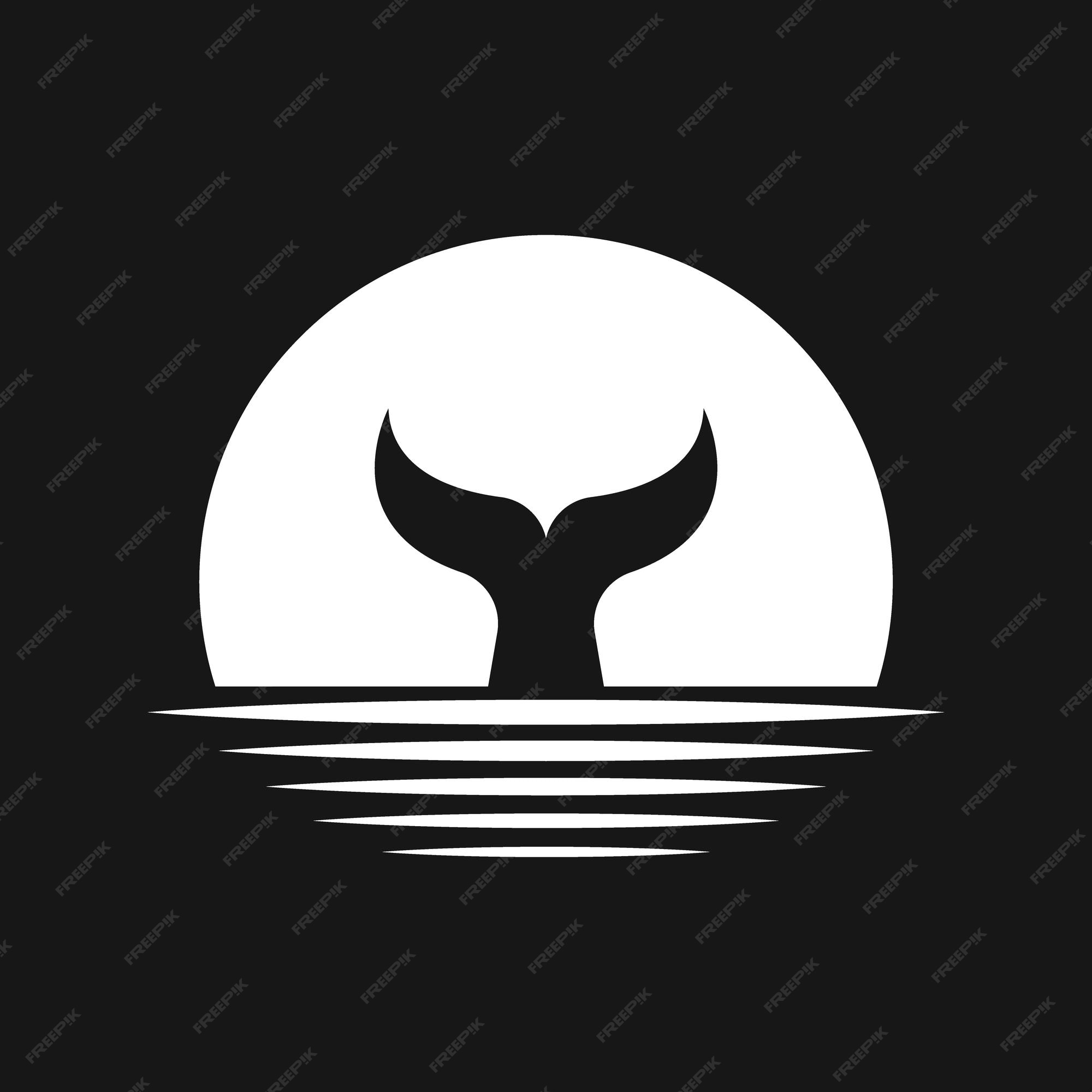The image is a detailed black and white drawing featuring a whale's tail against a black background. At the center of the illustration is a prominent white circle, likely representing the sun or the moon, which occupies roughly 40 to 50 percent of the image. Within this circle, a black silhouette of a whale's tail is prominently displayed. Below the tail, there are five white lines of varying lengths that probably signify water ripples, with the shortest at the bottom and the longest at the top. Scattered throughout the black background are repeating patterns of the word "freepik," adding a distinctive texture to the backdrop. This watermark text is consistently spaced and appears to be arranged in a sequence, contributing to the overall composition of the artwork.